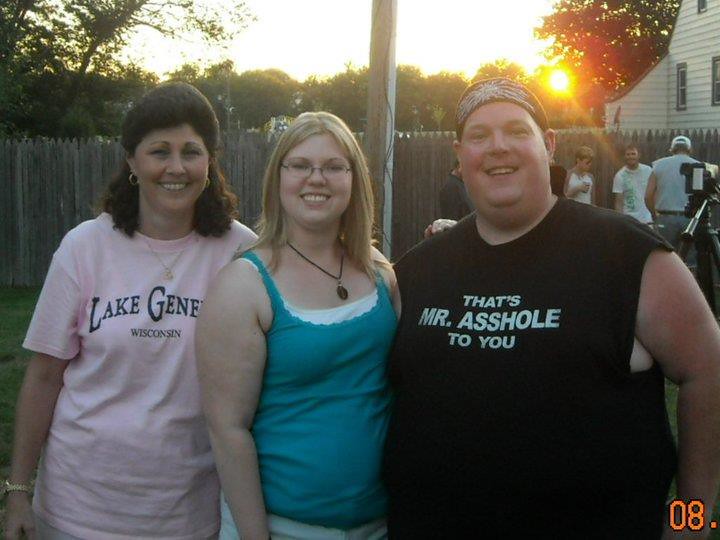This image captures a vibrant, outdoor family gathering, likely in someone's backyard, as the late afternoon sun casts a warm glow over the scene. In the foreground, three central figures pose for the camera. On the far right is a large young man with a round face, sporting a black bandana decorated with a white spider design, and a black muscle shirt with the phrase "That's Mr. Asshole to you." Standing next to him in the middle is a young girl with blonde hair, dressed in a blue tank top and wearing a black necklace. To her left is an older woman with thick brown hair, adorned with hoop earrings and a pink t-shirt that reads "Lake Geneva, Wisconsin." Behind them, a wooden privacy fence made of vertical brown planks stretches across the background, with a light pole and trees dotting the distant landscape. Additional people are gathered in the background, seemingly engaged in conversation or preparing a meal, enhancing the familial and welcoming atmosphere of this outdoor snapshot.